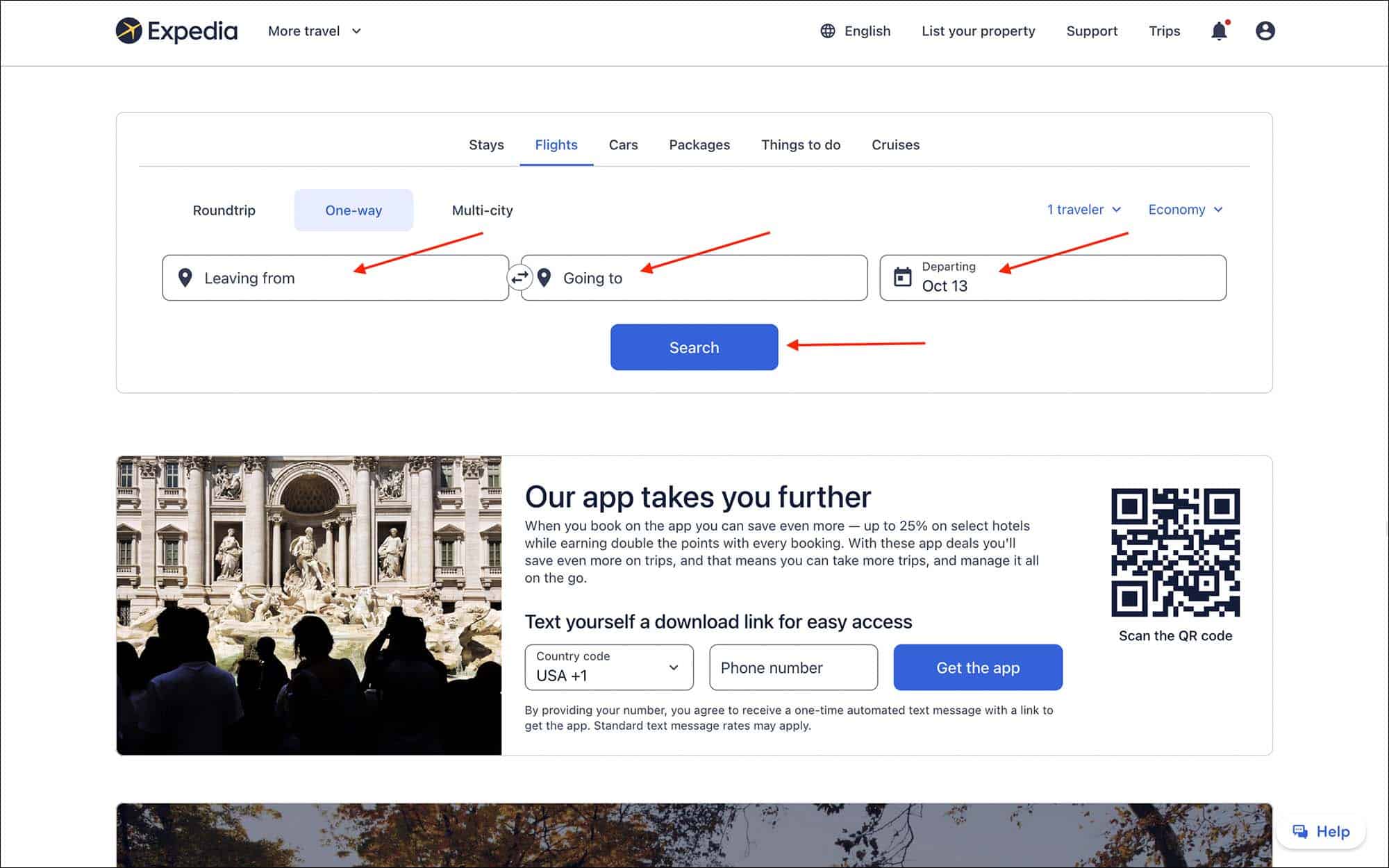This screen capture showcases the homepage of the travel website Expedia, with a predominantly white background. In the upper-left corner, the Expedia logo is visible, consisting of a black circle featuring a yellow plane. Adjacent to the logo is a pull-down menu labeled "More travel." 

In the top-right corner, various icons and links are displayed: a globe icon next to the English language setting, options to "List your property," access to "Support" and "Trips," a bell icon with a red notification dot, and a black circle with a white person icon. Below these, the primary navigation bar lists tabs for "Stays," "Flights" (highlighted in blue with an underline), "Cars," "Packages," "Things to do," and "Cruises."

Further down, the flight booking section begins with options for "Roundtrip," "One-way," and "Multi-city," with the "One-way" option highlighted in a light blue box. Red arrows point to relevant fields including "Leaving from" and "Going to," both with location pin icons, as well as "Departing," accompanied by a calendar icon and displaying the date "October 13." A section indicating "One traveler, economy" features a pull-down menu, with another red arrow pointing to a large blue and white "Search" button.

Beneath the booking section, an image depicts Renaissance-style gray statues and groups of people photographing them. Overlaying the image, black text states: "Our app takes you further. When you book on the app you can save even more up to 25% on select hotels while earning double the points with every booking. With these app deals you'll save even more on trips and that means you can take more trips and manage it all on the go."

The text further invites users to "Text yourself a download link for easy access," providing a field for entering a phone number prefixed by the country code "USA +1." A blue button labeled "Get app" and a black QR code with the instruction "Scan the QR code" are also present. At the bottom of the screen, there is a partial view of trees and a white box labeled "Help."